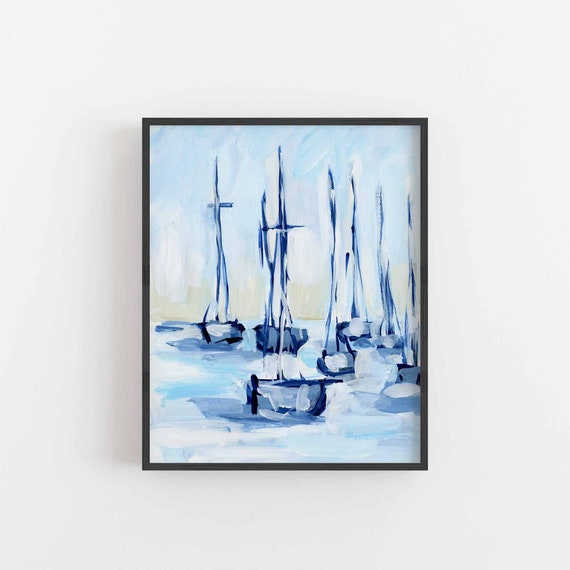This is a color photo of a painting on a white wall. The painting, enclosed in a thin black frame, appears to be executed with broad brush strokes, lending it a distinctly impressionistic quality rather than fine detailed work. The dominant color palette features mostly white, light blue, darker navy blue, and subtle hints of yellow and green. Depicted in the artwork are seven boats with tall white masts, positioned in a body of water characterized by light blue and darker blue hues, accented with white waves. The boats themselves are outlined with dark blue, making them stand out against the pale, almost snowy-looking water. The background seems to transition into a faintly colored sky, blending cream with pale blue, adding to the serene and somewhat ethereal atmosphere of the painting. The entire composition suggests an acrylic medium, capturing a snapshot of peaceful maritime scenery.